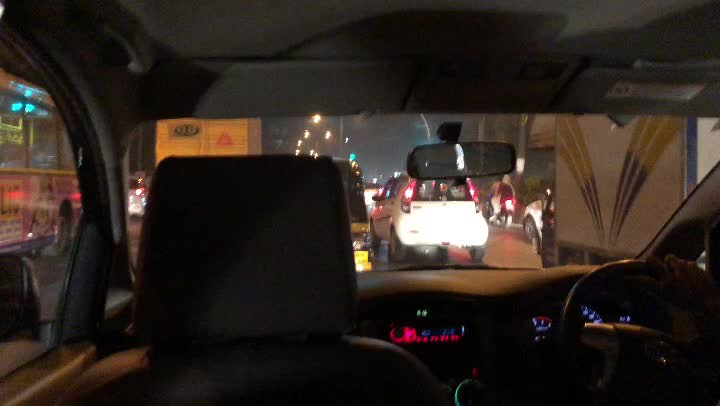This rectangular photograph, taken from the back seat of a vehicle, captures a night-time scene through the eyes of a passenger. The perspective reveals the dark interior of the car, with a black headrest dominating the foreground. To the right of this headrest, a black steering wheel rests on the right side of the car, indicating that this vehicle is likely from a British Commonwealth or former colony. The dashboard features a glowing speedometer and several illuminated buttons, adding a splash of red and dark blue light to the otherwise dimly lit cabin. Through the windshield, we see a congested road illuminated by streetlights and neon storefronts in the distance. Directly ahead, a white SUV with glowing brake lights is surrounded by various other vehicles, including a box truck on the right and another truck to the left, all seemingly stuck in traffic. This vivid scene showcases the interplay of interior vehicle lights against the backdrop of a bustling, brightly lit street at night.